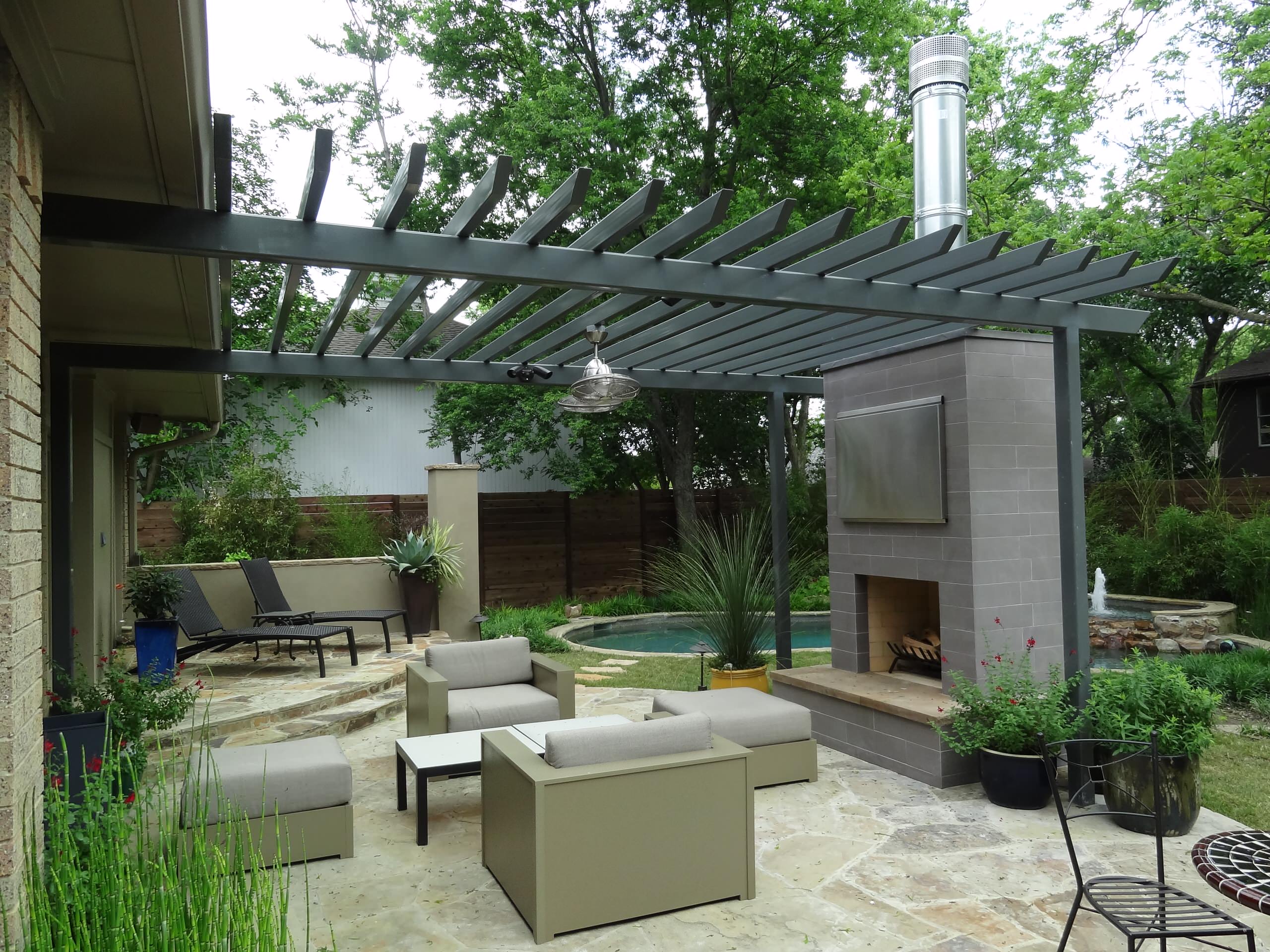The photograph captures a luxurious outdoor patio area, highlighting a backyard oasis. The focal point is a stylish canopy constructed with dark gray wooden slats forming a roof. Hanging from the canopy is a combination light fixture and fan, illuminating the elegant setting below. Nestled under the canopy is a cozy arrangement consisting of a table flanked by two chairs, two stools, and additional seating including a couple of couches and cushions. This setup rests atop a stone tile floor. One prominent feature is the outdoor fireplace composed of gray brick, complete with a chimney and an exhaust fan. 

Surrounding the patio are several planters filled with vibrant, flowering plants, adding bursts of greenery and color. Adjacent to the patio is a pool, bordered by a grassy yard and complemented by a fountain on the right side. Further enhancing the scene are two black lounge chairs and a blue and brown planter, each holding lush plants. A wooden boundary wall modestly encloses this outdoor sanctuary, connecting subtly to the main house visible on the left edge of the image.